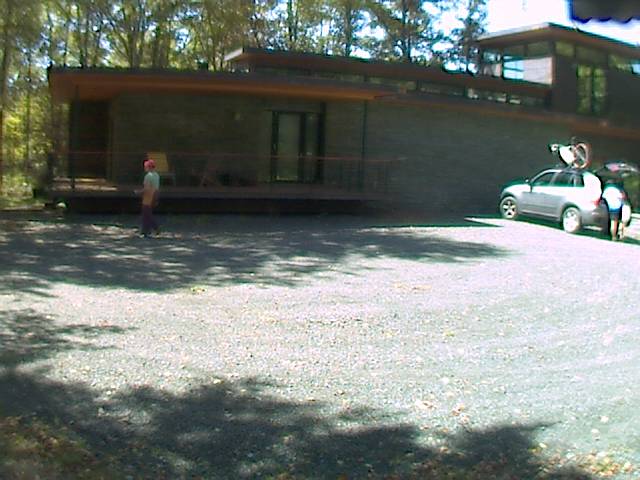In the captured daytime image set outdoors, the background features a dense array of tall, green trees with glimpses of a light blue sky interspersed among the leaves. A three-story building with gray stone walls and flat brown roofing stands prominently beneath the trees. The building's facade is punctuated by numerous glass panes adorned with black trimming. The bottom level has a brown balcony featuring a glass door with black trimming and two chairs – the leftmost chair is yellow, and the rightmost chair is a reddish-brown. 

In front of the balcony, a person is walking to the left, dressed in a red hat, a blue shirt, and purple pants, with their left arm flexed at the elbow. To the right, a silver car with an open trunk and a bicycle mounted on the roof is visible. Another person, clad in a blue shirt and black shorts, is reaching into the trunk, holding a white object in their right hand. The ground is covered in gravel with brown patches and shadows of the trees cast upon it.